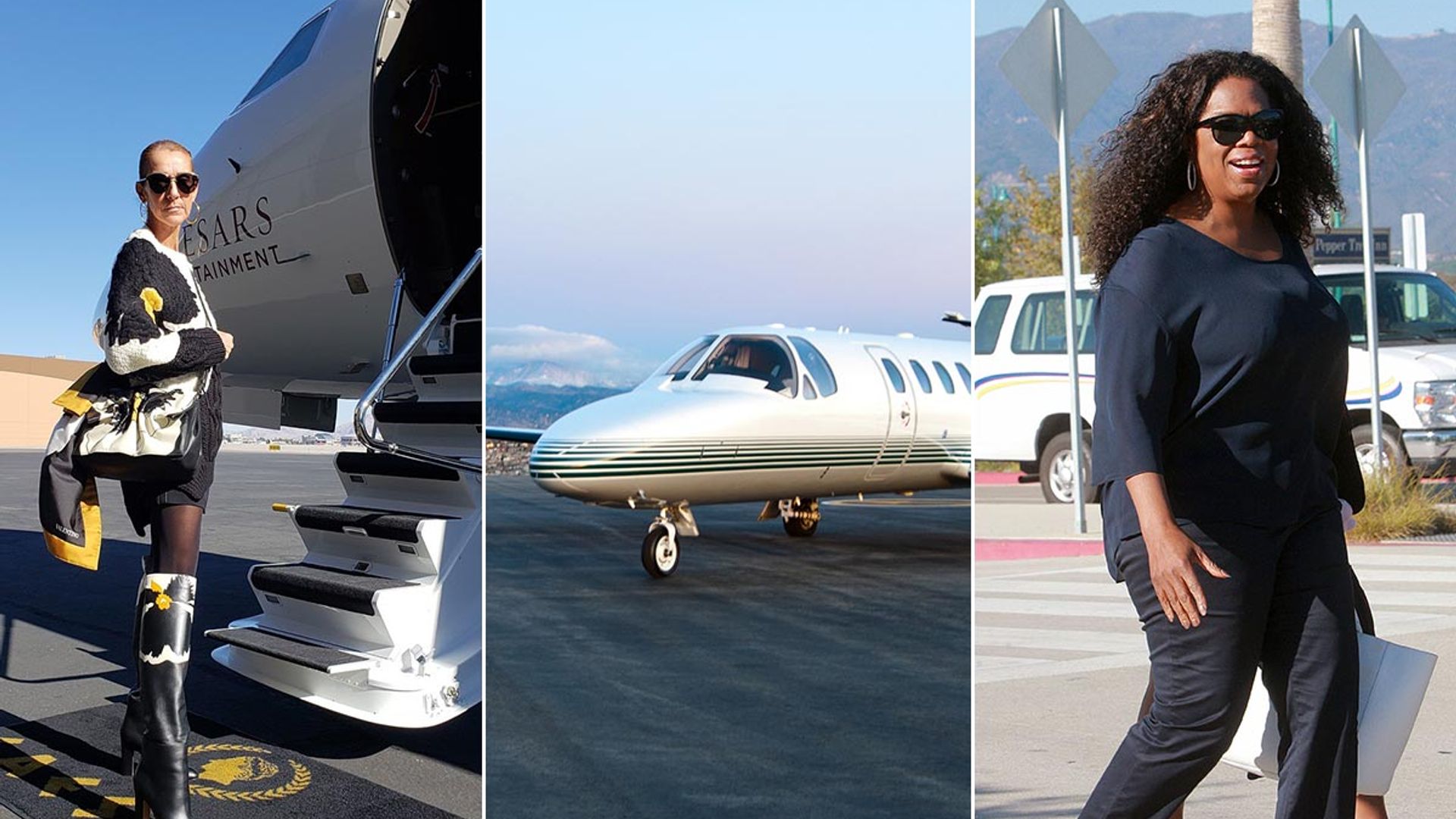The image is a horizontally formatted, color triptych comprising three distinct photographs. The left photo features Celine Dion standing confidently in front of a private jet with "Caesars Entertainment" emblazoned on its nose. She is poised to board, standing on a mat with the "Caesars Palace" logo partially visible. Celine is dressed in a coordinated black and white ensemble that includes knee-high faux cowhide and black leather boots, a matching jacket, and a purse with gold accents. She accessorizes with long hoop earrings and sunglasses, and her short hair complements her serious expression as she looks into the camera.

The middle photo focuses solely on the front of a sleek private jet, possibly a Learjet, positioned on a runway with distant mountains providing a scenic backdrop. 

The right photo captures Oprah Winfrey strolling on a sunny day. She wears sunglasses, a dark shirt with three-quarter sleeves, black pants, and hoop earrings. She carries a white shopping bag in her left hand and smiles warmly. Behind her, a minivan or SUV is parked, with mountains and some indistinguishable signs in the background.